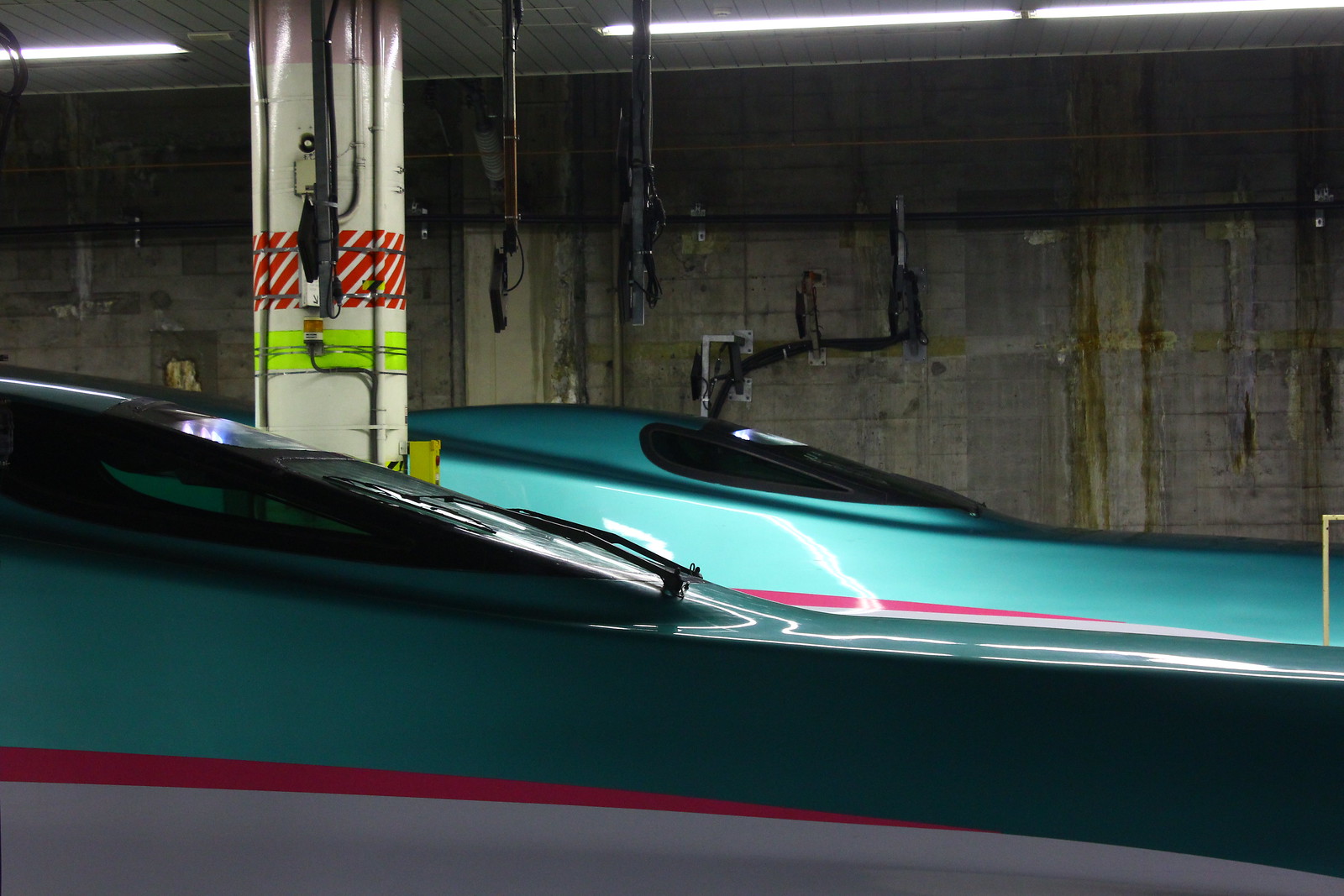This photograph captures the interior of an unfinished garage with a distinctly industrial feel. The room features concrete brick walls, heavily stained with a mossy brownish-green discoloration, and a roof constructed of tiled panels in a horizontal pattern, primarily white but showing signs of wear. The ceiling is equipped with long, rectangular fluorescent lights that provide stark, bright illumination throughout the space. Hanging down are black poles that appear to carry electrical cords or wires.

In the center of the garage, prominently positioned beneath the lights, are two large vehicles that draw the eye with their striking color scheme. These vehicles have a teal metallic green body, accented by a hot pink stripe, and a white lower section. The windshields are notably slanted and heavily tinted, almost horizontal in appearance, and equipped with windshield wipers.

Separating the two vehicles is a prominent cemented post adorned with multiple bands of tape: a fluorescent green band and a red-and-white striped band. This post also supports various wires and conduits that contribute to the unfinished, utilitarian atmosphere of the space. The overall scene is one of stark contrasts, with the bright lights accentuating the grime and industrial features of the garage.